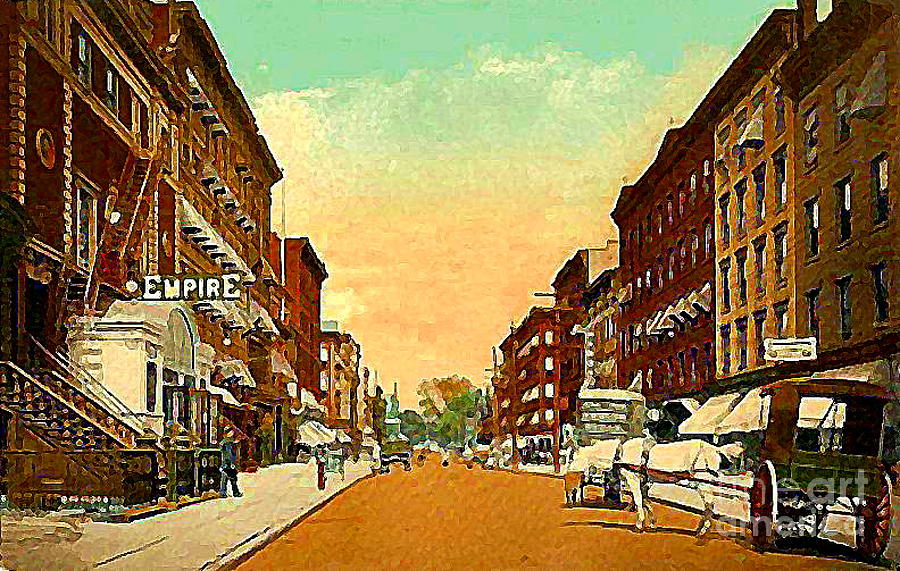This image is a slightly blurry, colorful painting depicting a historic city street scene. The image captures four to six-story buildings with uniform rows of windows, flanking both sides of a dirt road. On the left side, a prominent white-lettered sign reads "Empire" above a storefront with an archway and stairs, giving the building an office-like appearance. On the right, a white horse pulls a brown and green carriage with large old-fashioned wheels, situated near the bottom corner of the image. Sidewalks line both sides of the street, dotted with a few pedestrians, including a man exiting a building on the left. The painting skillfully narrows the street perspective, leading the viewer's eye toward the distant trees and a serene, light blue sky transitioning into a pink-orangey sunset.